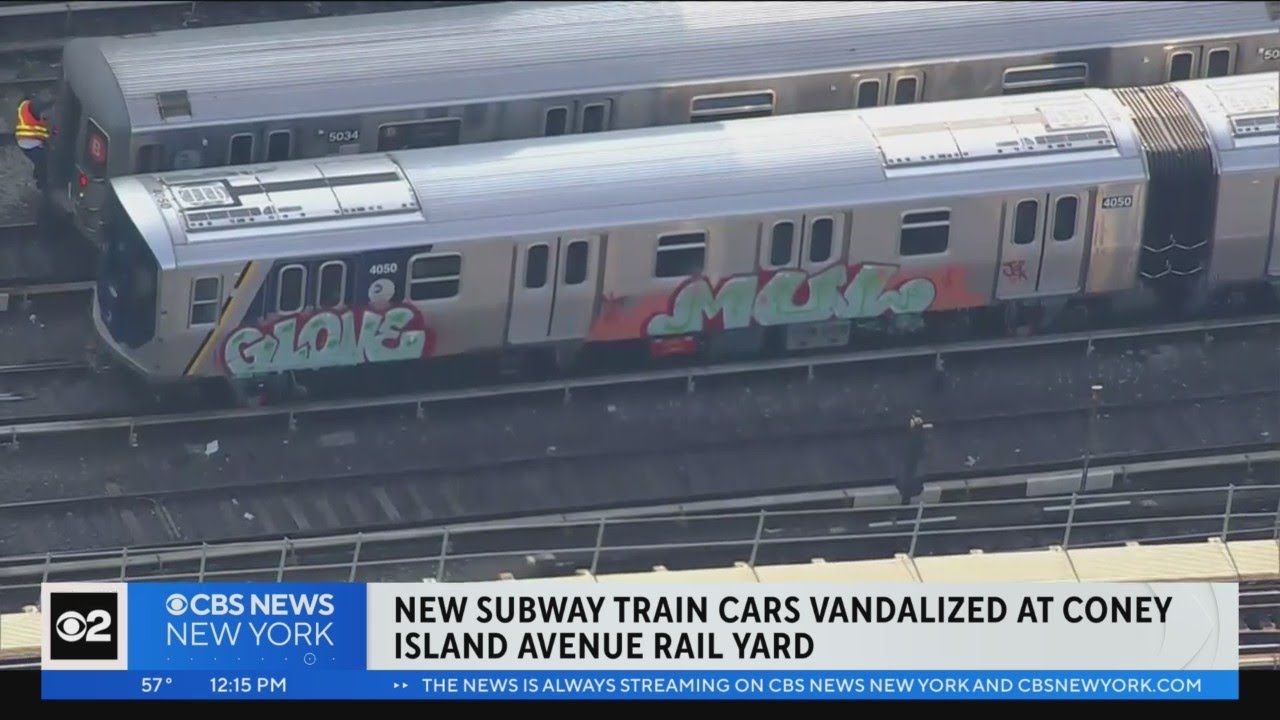This detailed still image, captured from a CBS News New York broadcast, shows two new, shiny silver subway train cars situated on train tracks at the Coney Island Avenue railyard. The broadcast banner at the bottom of the image features the CBS News New York logo and a headline stating, "New Subway Train Cars Vandalized at Coney Island Avenue Railyard," along with a temperature of 57 degrees and a timestamp of 12:15 p.m. The news is also streaming on CBS News New York and cbsnewyork.com.

The overhead view reveals graffiti on the train car positioned in front. On the left end of this train car, the graffiti consists of large green bold letters with a red outline spelling "glove." To the right, another stylized piece of graffiti appears, likely containing the letters "M," "U," and an indeterminate letter, similarly rendered in bold green text with a red and possibly purple background. The train cars' polished, reflective surfaces highlight their newness despite the evident vandalism.